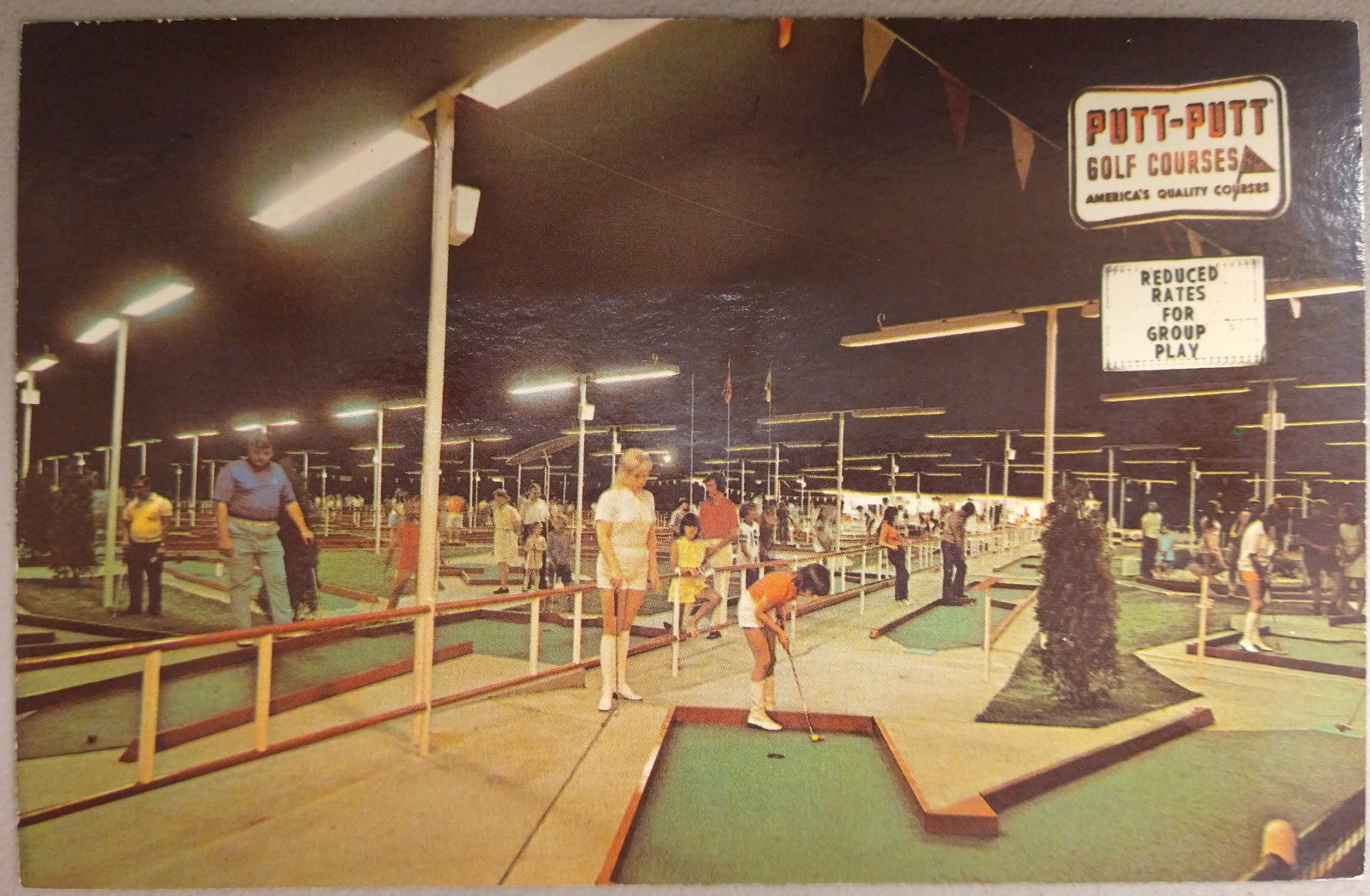This vibrant yet nostalgic photograph captures a lively outdoor miniature golf course, likely dating back to the late 70s or early 80s, evident from the faded tint and clothing styles. The scene is set at night, illuminated by rows of overhead lights strung across the course. In the upper right corner, a brightly lit sign proclaims "Putt-Putt Golf Courses, America's Quality Courses" in bold red letters, accompanied by a changeable message board announcing "Reduced Rates for Group Play."

At the heart of the image, artificial green turf spreads out, dotted with various miniature golf holes. A person, hunched in concentration, is about to putt; they wear an orange shirt, white shorts, and matching white boots. To their left stands a woman dressed similarly in a white short-sleeved shirt, white shorts, and white boots. The attire and overall vibe suggest a bygone era, rich with the charm of past fashion trends. Adding to the festive atmosphere, red flags hang from strings across the top of the photo. The image, bordered in a faint brown, exudes a sense of communal fun and timeless leisure.